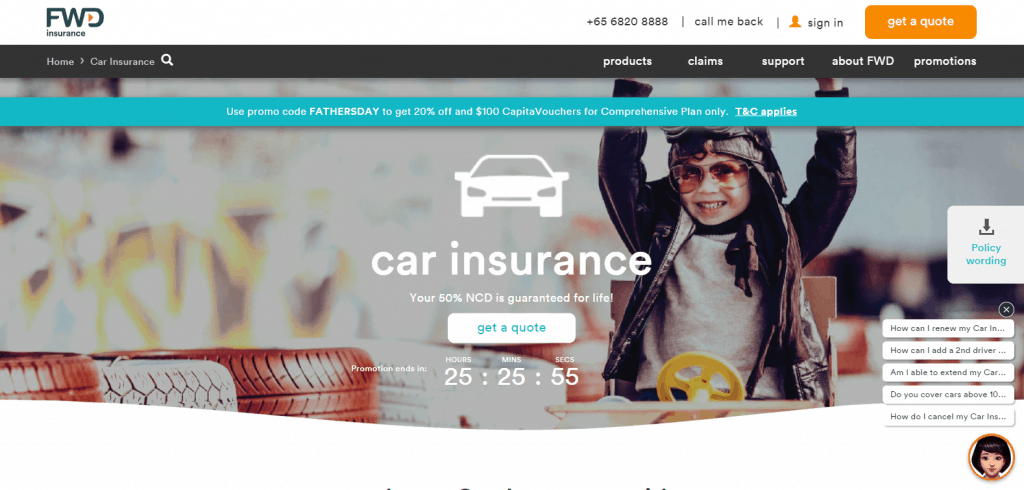This screenshot captures the homepage of the FWD Insurance website. The top section features a prominent white banner. Positioned in the top-left corner is the FWD logo, with the letter "D" creatively integrated with an orange arrow, followed by the word "Insurance" in a sophisticated dark green font. On the right side of the banner, there is a customer service phone number, a "Call me back" option, a "Sign in" button accompanied by a small orange avatar, and an eye-catching orange button with rounded corners that prompts users to "Get a Quote."

Beneath the white banner lies a sleek black navigation bar. The left side of this bar offers quick links to "Home" and "Car Insurance," along with a search icon for easy access. The right side of the navigation bar provides links to various sections such as "Products," "Claims," "Support," "About FWD," and "Promotions," all in crisp white text.

The heart of the homepage is dominated by a charming image of a young boy donning an old-fashioned pilot's hat, whimsical aviator goggles, and a white shirt. He is seated in what appears to be a homemade go-kart, navigating around tires, exuding a sense of playful adventure. Superimposed on this engaging background is a white graphic of a car, bearing the text "Car Insurance" and a "Get a Quote" button. A countdown timer below it announces the promotion's end in 25 hours, 25 minutes, and 55 seconds.

To the right of the main imagery, there is a chat support option, featuring a cartoon profile of a woman with black hair. This chat feature offers quick interaction buttons for five pre-set messages, facilitating immediate customer service assistance.